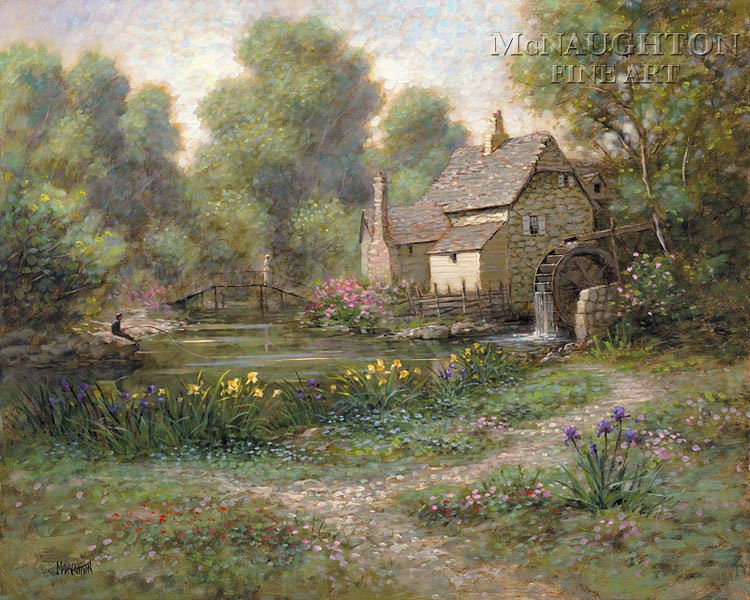This detailed impressionist watercolor painting, signed "McNaughton Fine Art" in the bottom left corner, features a serene old French countryside scene. The focal point is a charming stone cottage with a sloped roof and three distinct levels, adorned with wood paneling in some sections and two chimneys protruding from different areas. Set against a backdrop of lush trees and a whitish-blue sky, the cottage also boasts a spinning wooden water wheel at its back, with water cascading down.

In the foreground, a vibrant array of flowers flourishes, including purple irises, yellow daffodils, and pink blooms, creating a lively palette of colors. Among these flowers, a cobblestone path, intricately painted with whites, grays, and browns, winds through the grass leading up to the cottage. 

To the right, a pond stretches out with a delicate wooden bridge arching over it. A man can be seen crossing the bridge towards the pink flowers directly in front of the house. On the left-hand side of the pond, a little boy is depicted intently fishing in the tranquil waters. The scene is encircled by a stone fence, further enhancing the rustic charm of this picturesque countryside retreat.